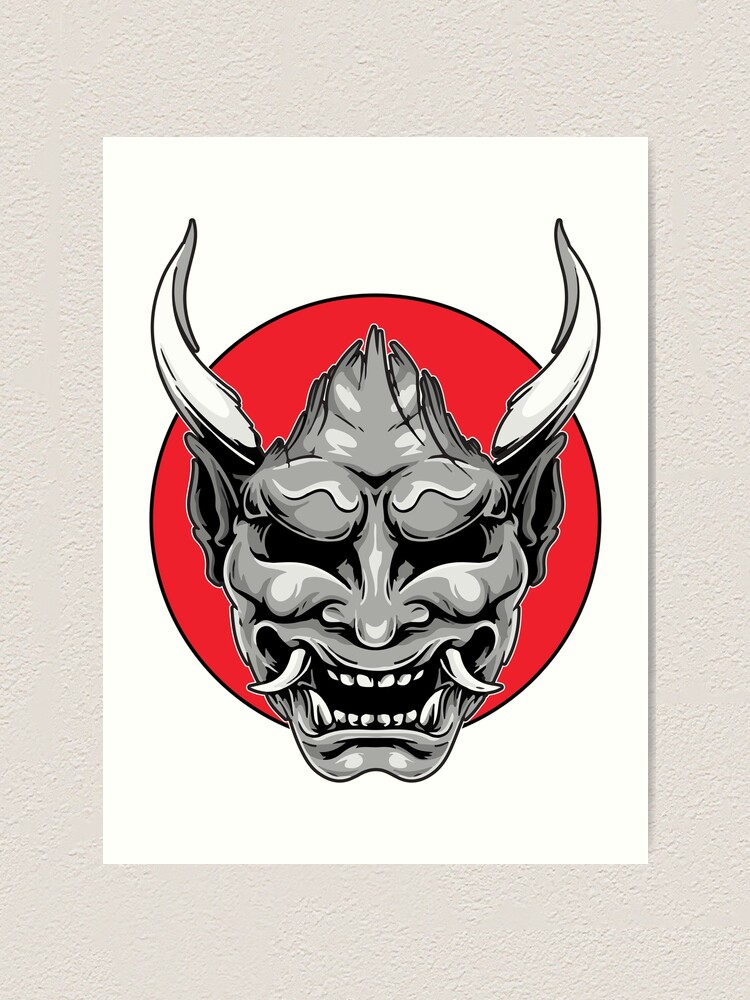The image depicts a vertical rectangular area, likely a textured beige wall, with a white A4-sized piece of paper or poster affixed to it. The illustration on the paper features a striking red circle, reminiscent of the Japanese flag, serving as the backdrop for a grotesque, demonic face. This face appears to be a disturbingly detailed yet cartoonish rendition, merging elements of human and mythical demon characteristics. 

The demonic figure has a scrunched, gray face with two white, jagged horns protruding from its head. It boasts large, pointy ears reminiscent of an animal, perhaps a wolf. The top of its head is pointed, possibly covered in hair, adding to its menacing appearance. The eyes are either hollow or solid black, with pronounced brow ridges above them. Emphasizing its horrific expression, the creature has a wide, gaping mouth filled with a mix of human-like teeth and prominent, outward-jutting fangs. The entire composition, with its textured background and eerie subject, creates a visually arresting and unsettling scene.